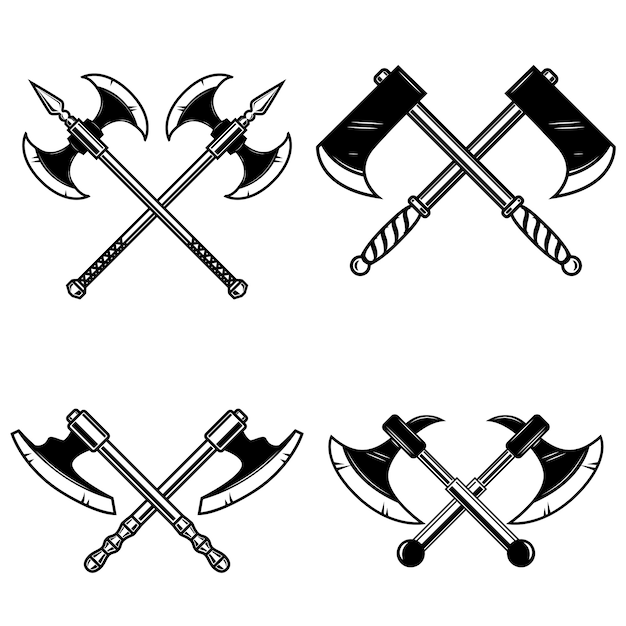The image is a black and white composite featuring four separate pairs of animated axes, each pair arranged in a crossed configuration. The top left pair features double-sided axes with spear-like points protruding upward, complemented by patterned handles near the hilt. Adjacent to it on the right, another pair showcases single-sided hatchets with sharp, curved blades and rounded handles. Below, the bottom left pair displays similar single-sided hatchets, but with a more pronounced curvature and larger round ends on the handles. The bottom right pair mirrors the bottom left but lacks any design patterns, presenting a flat handle. All axes, distinct in shape and design, are rendered in an illustrative, computer-generated style, emphasizing their sharpness and detailing through monochromatic tones.